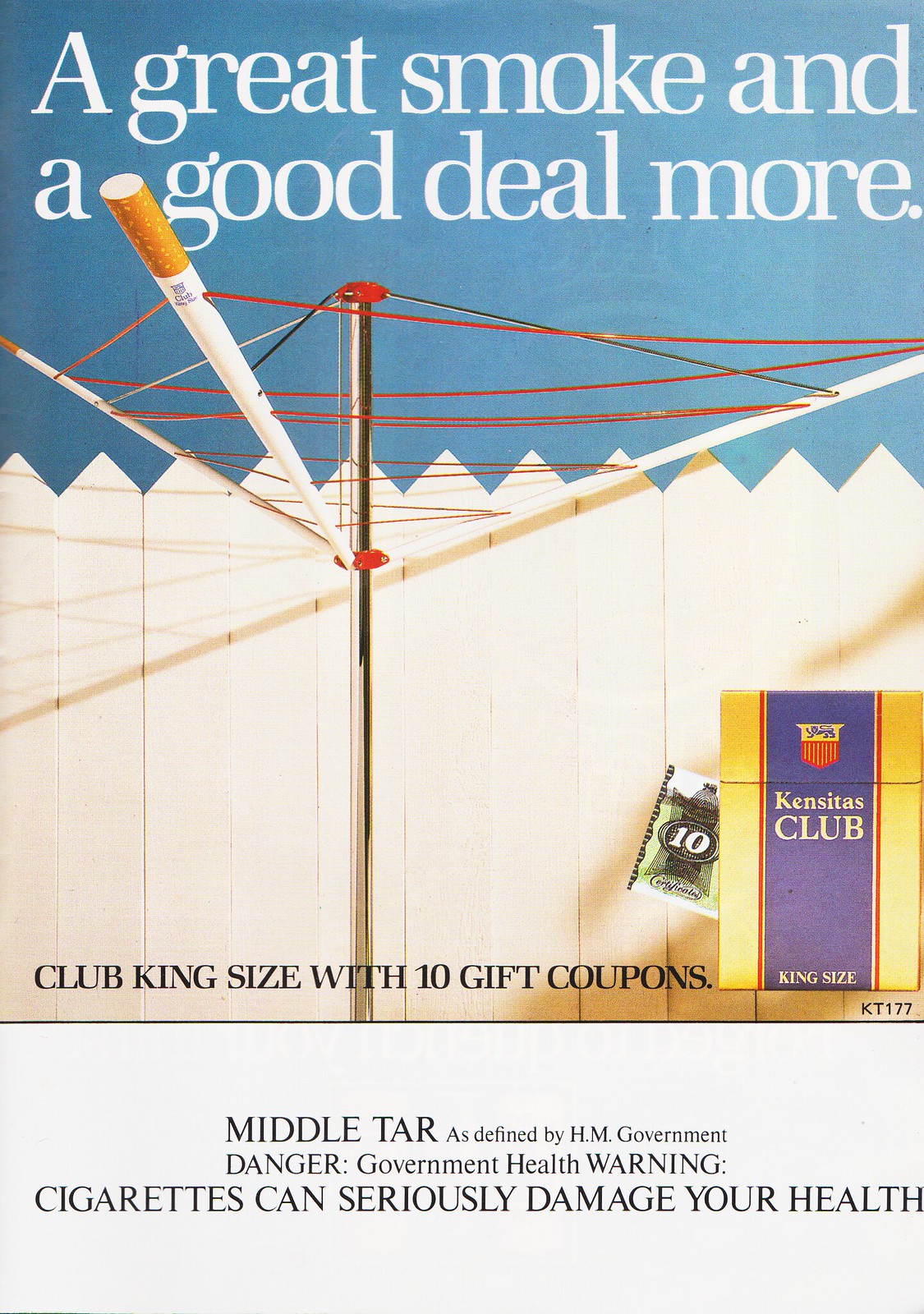The advertisement displays a vibrant scene centered around a Kinsita's Club King Size Cigarettes pack. The packaging of the cigarettes features a gold and purple color scheme with a distinctive red stripe and black text on a gray banner at the bottom. Dominating the background is a picturesque white picket fence, reminiscent of suburban tranquility, under a crisp light blue sky. 

In the foreground, a laundry hanger has been creatively transformed; its upper bars are replaced with cigarettes. Above this inventive display, large white text reads, "A great smoke and a good deal more." Below, black text emphasizes "Club King Size with 10 gift coupons." Additional small print indicates, "middle tar as defined by HM government," along with a stark health warning: "Cigarettes can seriously damage your health." This detailed and visually impactful advertisement not only promotes the cigarette brand but also blends elements of everyday life with the product, encasing the promise of luxury and convenience in an artful suburban setup.